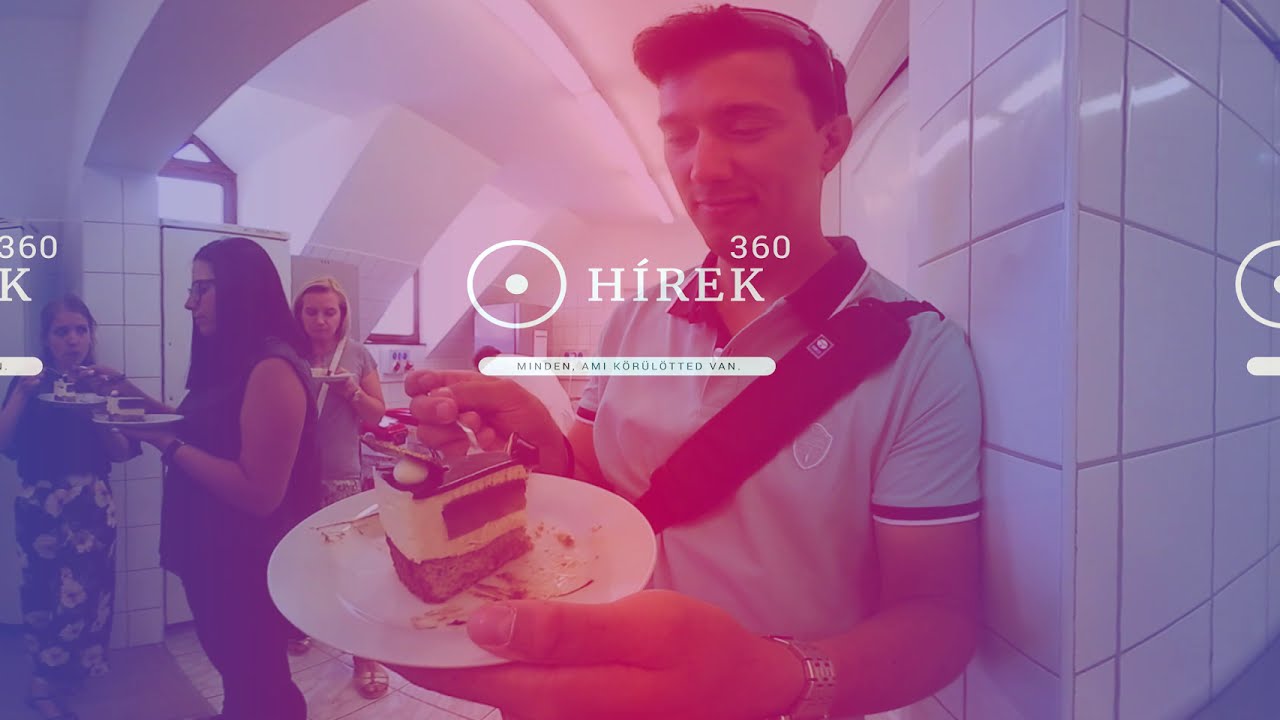The image, a horizontally aligned rectangular photograph with somewhat muted colors, appears as a faded screenshot of a website or interactive experience. It depicts a slightly blurry scene in a kitchen, where white tiled walls with gray grout form the background. Central to the image is a young man, possibly in his 20s, standing near the tiles and staring down at a plate he holds in his left hand with a fork in his right. The plate contains a slice of multi-layered cheesecake topped with chocolate. The man has short black hair with sunglasses perched on top of his head, and he is dressed in a light blue polo shirt with a white logo on the chest and a dark blue collar. A black strap, presumably from a shoulder bag, is slung diagonally across his chest from his left shoulder. He appears to be smiling subtly, perhaps in anticipation of eating the cake. 

To the left in the background are three women, each holding similar plates with slices of the same cake. One woman, visible from the side, wears a sleeveless black top and black pants. Another, farther to the left, dons a black blouse paired with a long floral skirt. The third is seen partially due to the man's plate obstructing the view; she has a short-sleeved gray top. 

Overlaying the central portion of the image is a circular logo with a white dot inside, accompanied by the text "HIREK 360" in white, contributing to the appearance of a digital interface.